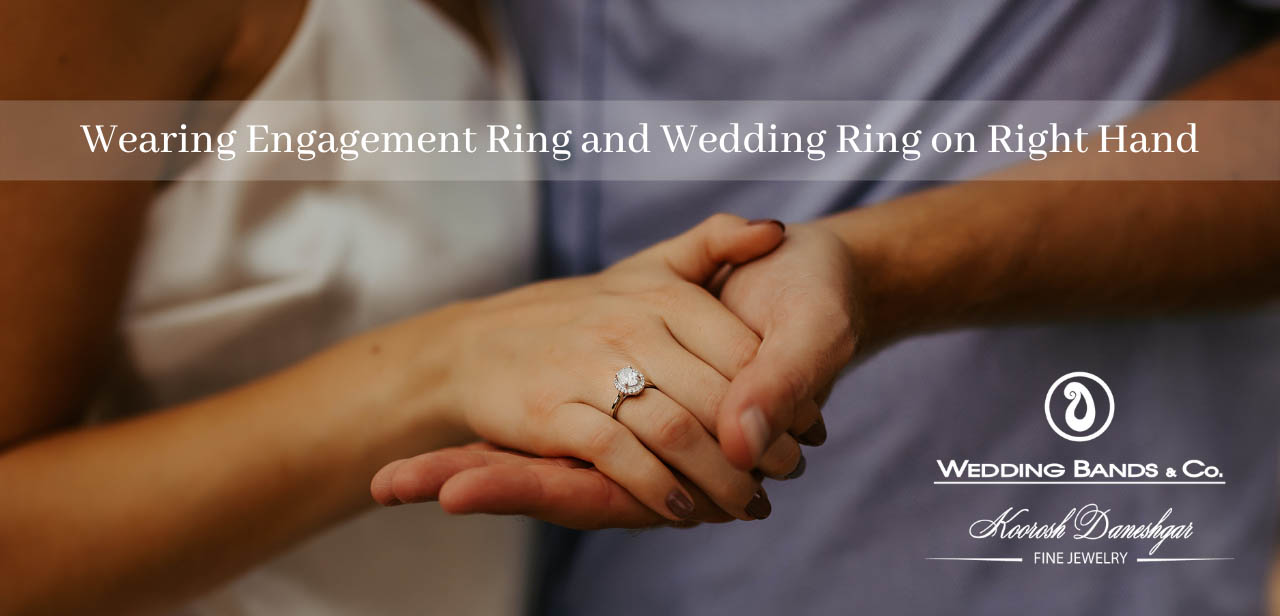This advertisement for a wedding jewelry store prominently features the clasped hands of a man and a woman. The woman’s hand, adorned with a large diamond engagement ring on her ring finger, is positioned on the left. She has dark red nail polish and is dressed in a sleeveless white shirt or gown, visible from the chest down. The man’s torso, attired in a blue or purple t-shirt, is seen on the right. The background is slightly blurred, drawing focus to their interlocked hands.

A white banner across the top of the image displays the text, "Wearing Engagement Ring and Wedding Ring on Right Hand." In the lower right corner, a white logo features a distinctive teardrop design, accompanied by the text, "Wedding Bands and Company, Kurosh Daneskar, Fine Jewelry." The intimate placement of the couple and the detailed emphasis on their rings highlight the elegance and romance associated with the jewelry being advertised.